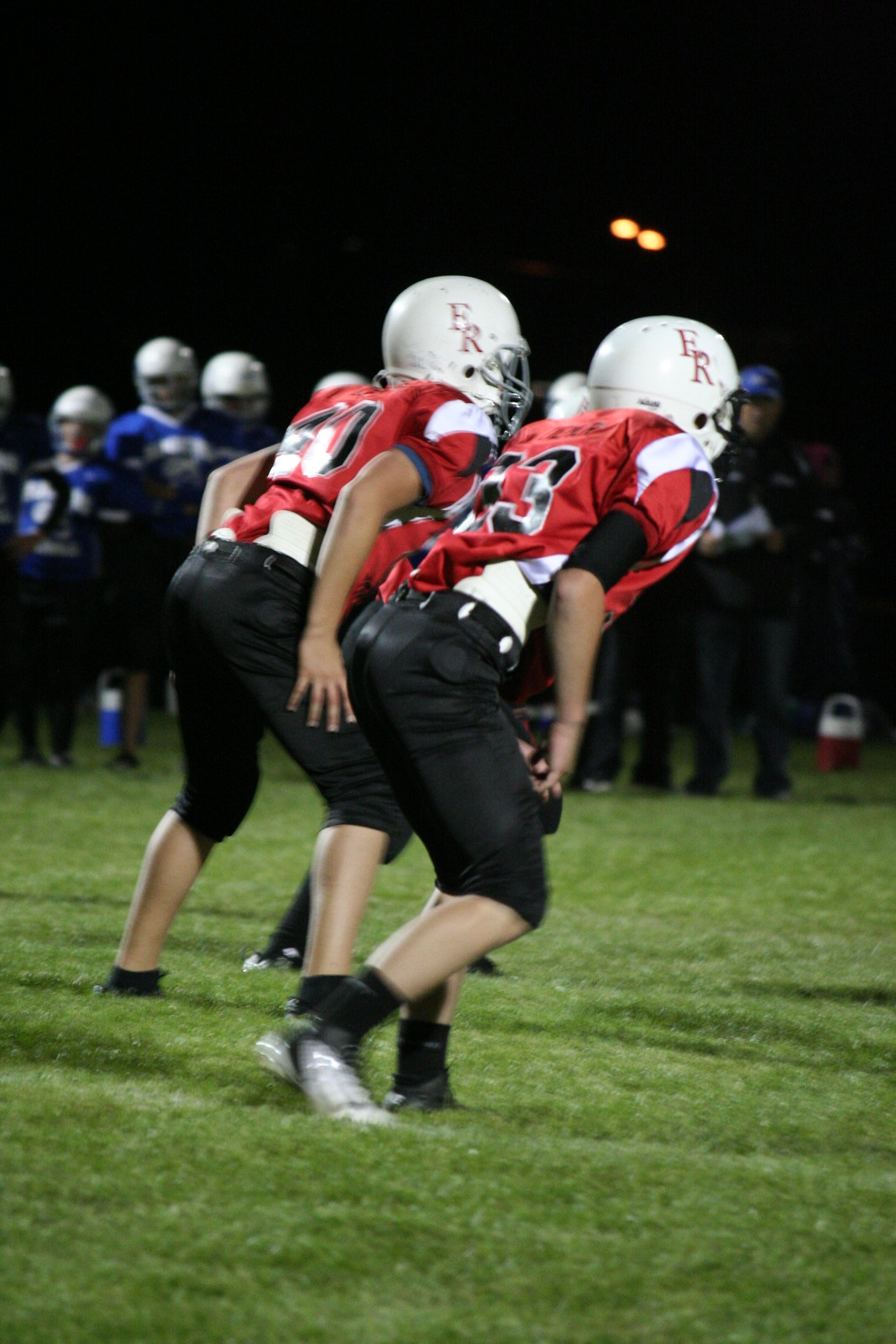This image, taken at night during what appears to be a high school football game, captures a compelling scene on the field. The backdrop is a completely dark sky, illuminated only by a distant streetlight casting a dim yellow glow. The green turf field is prominent, suggesting a soft, well-maintained surface. Central to the image are two high school-aged football players, both crouched in ready-to-run stances. They wear white helmets with red "FR" lettering, red jerseys with black numbers (although the numbers are not legible), black football pants, black socks, and gray or black shoes.

In the background, a team in blue jerseys with silver helmets and black pants stands on the sidelines. Additionally, there's a coach on the far right in a black jacket and pants. Near the sidelines, a large red water jug with a white top is visible. The softly lit field, blurred figures, and visible shadows add a sense of atmosphere and motion to this dynamic night game scene.